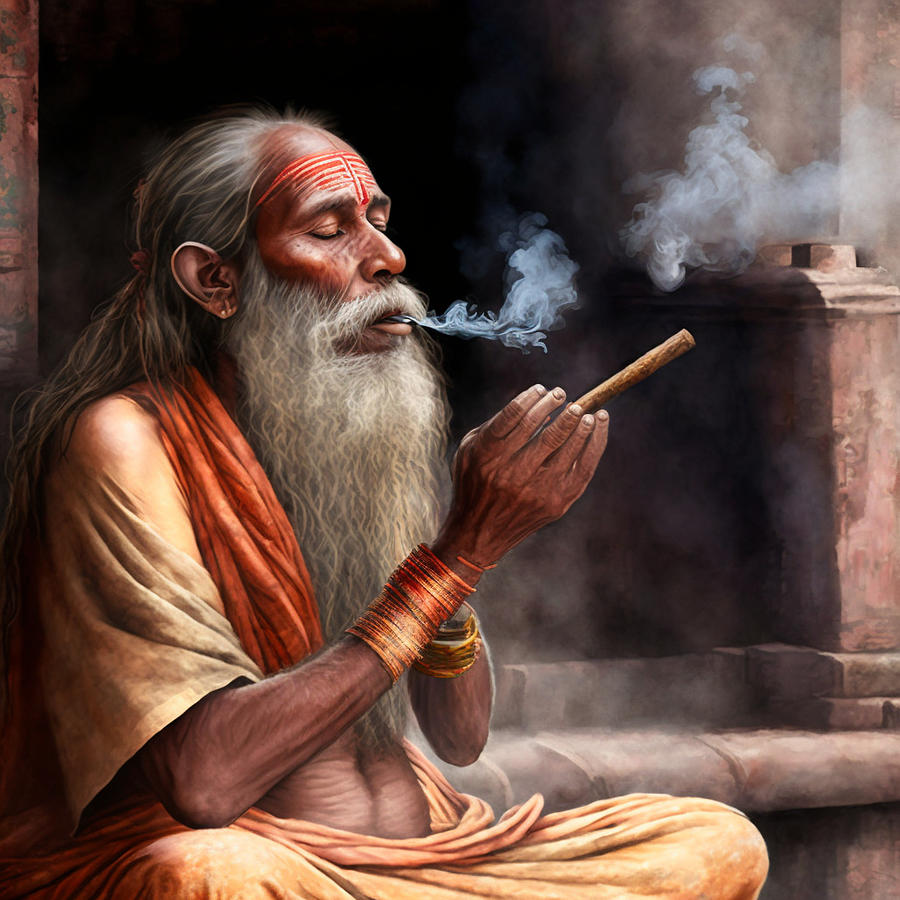An AI-generated image depicts an elderly man who appears to be meditating. The man, with his long grey beard reaching down to his belly button and equally long grey hair tied back, sits in a traditional cross-legged position, evoking a sense of tranquility and spirituality often associated with ancient tribes or sages from the Middle East or South Asia. He is dressed in a yellow robe paired with yellow pants and an orange scarf around his neck. His forehead is adorned with distinctive face paint: a red mark with orange and white horizontal stripes and a singular line running down between his eyebrows, adding to his mystic appearance.

The man is seen holding a cigar-like object in his left hand, from which trails of smoke wisp around him, contributing to the ethereal atmosphere of the scene. He has a bracelet on each wrist—gold on the right and bronze on the left. Additionally, the image contains some anomalies, such as the presence of six fingers on one hand, further indicating its AI-generated nature. The background is dark, enhancing the vividness of the smoke and the intricate details of his attire.